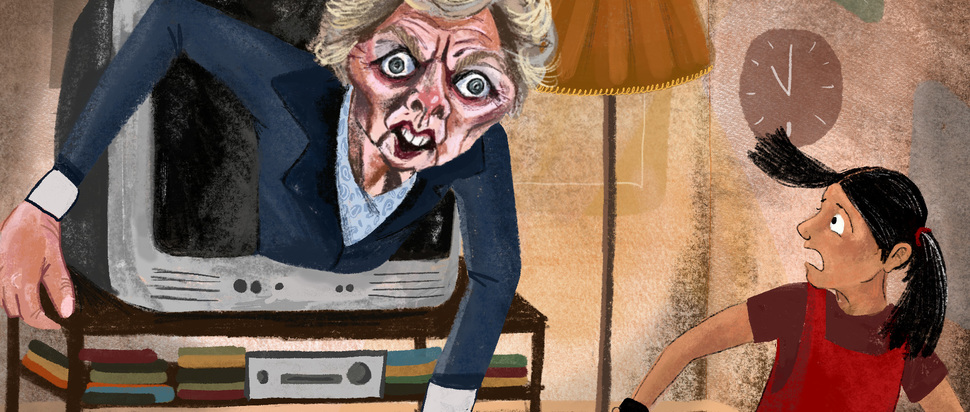This image is an eerie, cartoonish illustration that blends horror and surrealism. It depicts a young girl in a living room, standing before a TV with a look of sheer terror on her face. Her attire consists of red overalls over a t-shirt, and her black hair is styled in pigtails. Her mouth agape and eyes wide with fright, she stares in horror at the grotesque figure emerging from the television.

The figure appears to be a caricature of Theresa May, the former British Prime Minister, characterized by exaggerated features including large eyes and large teeth. She is depicted with gray, short hair and is wearing a blue pantsuit top. Her upper body protrudes menacingly from the TV screen, with her hands reaching out as if attempting to climb out of the device. Her appearance is both monstrous and nightmarish.

The setting includes a clock on the wall showing the time as approximately 10 o'clock and a lamp with an orange lampshade. The entire scene has a squashed and cropped feel, as though it has been extracted from a larger image; the top of the woman's head is cut off, and the young girl appears squeezed into a corner of the room. The overall composition adds to the unsettling atmosphere, making it unclear whether this is a moment of terror unfolding or a scene from a twisted dream.